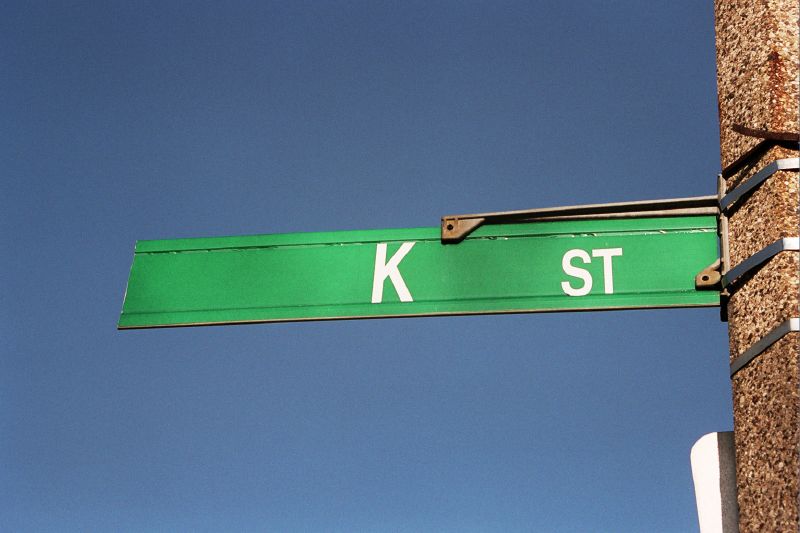The image features a crisp and clean green street sign in the foreground, prominently labeled in white with "K" at the center, followed by "ST" towards the right, indicating "K Street." The sign is mounted on a thick, rectangular stone pole, which exhibits a rocky texture with visible sediments. This pole is secured by three metal braces that wrap around it, ensuring the stability of the sign. The photograph is taken from a low angle, looking upward, which highlights the clear blue sky in the background with no visible clouds, suggesting a bright midday setting. The overall image quality is excellent, with sharp details of both the sign and the pole.